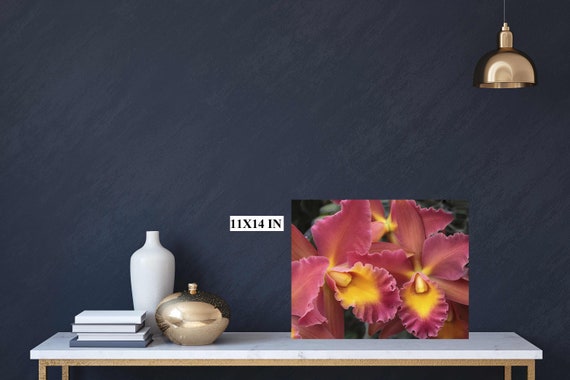The photograph captures an indoor setting featuring a rectangular white marble-topped table with gold-colored metal legs, placed against a gray textured wall. On the tabletop, starting from the right, there's an 11 by 14-inch printed picture of pink orchids with yellow and purple centers, showcasing the petals and the flower's core in a close-up view. Beside it, to the left, sits a shiny gold container with a lid and a central knob. Further to the left, a tall, narrow-necked, solid white vase is prominently displayed. In front of the vase, a neat stack of four nondescript books with white or grey spines is positioned. Overhead, in the top right corner of the image, hangs a pendant gold dome lamp, adding a touch of elegance to the composition.